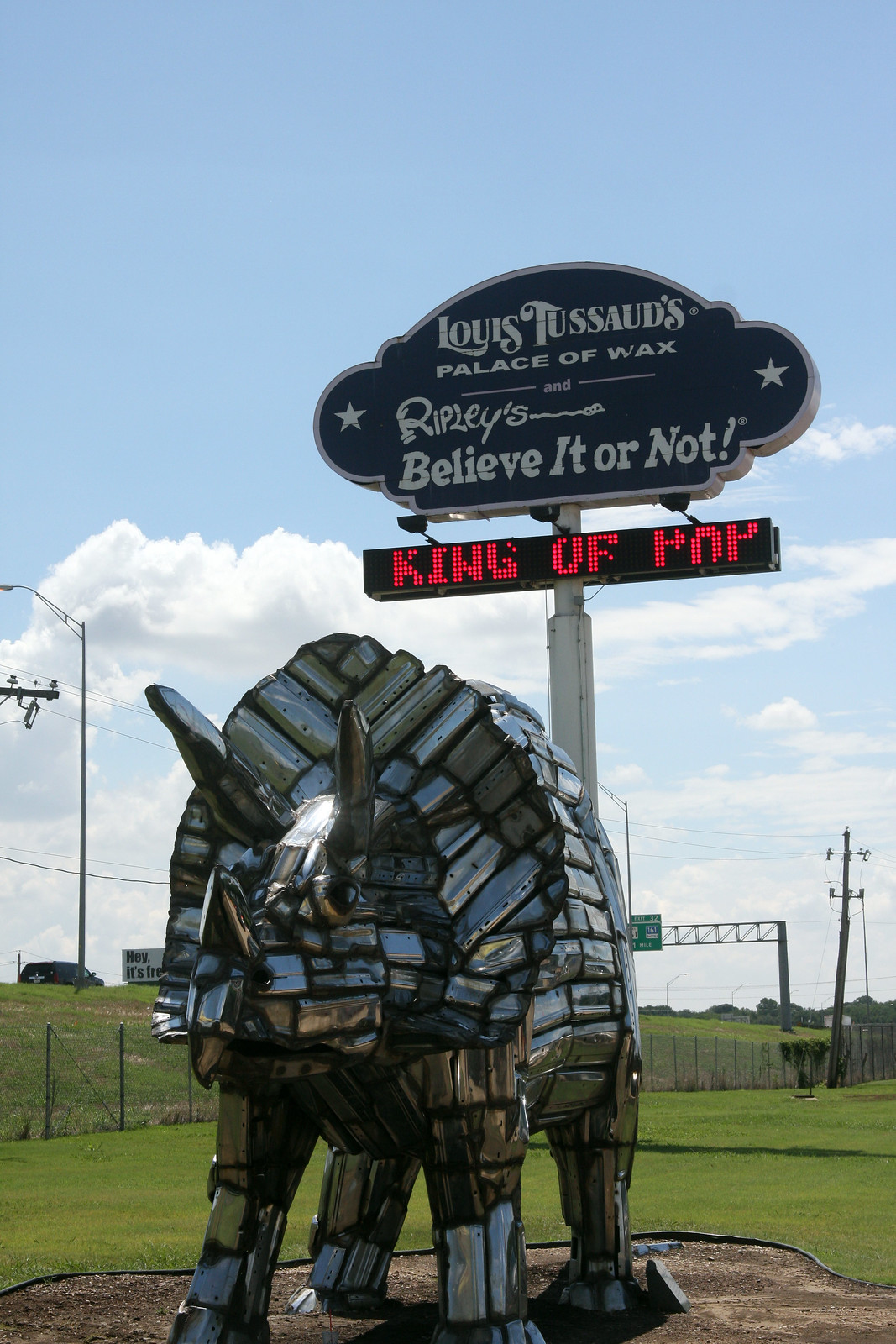This detailed image captures a striking outdoor scene featuring a low-angle shot of a large, intricately crafted sculpture of a Triceratops dinosaur. The dinosaur, approximately 8 feet tall, is constructed from various metal pieces, including what appears to be pipes, mufflers, and other car parts, giving it a shiny, chrome-like appearance. The sculpture is situated in a gravelly area adjacent to a well-maintained grassy patch. 

In the background, a prominent navy blue sign reads "Louis Tussaud's Palace of Wax" and "Ripley's Believe It or Not" in white letters, with an LED display beneath that says "King of Pop" in red letters. The sky is a vivid blue with scattered white clouds, and further behind, one can see a highway with indistinct signage and a few car sightings, along with power poles, indicating the proximity to a busy road. This roadside attraction evokes a nostalgic charm, characteristic of Louis Tussaud’s wax museums and Ripley's Believe It or Not establishments.